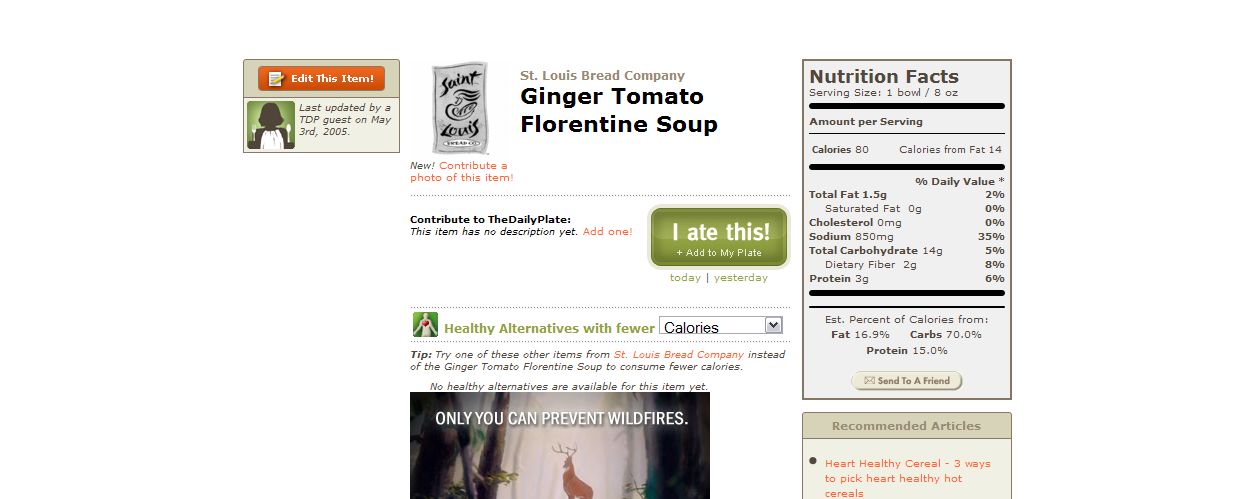This image depicts a screenshot from an old webpage, primarily showcasing a recipe for "Ginger Tomato Florentine Soup" from the St. Louis Bread Company. The website features an orange button in the upper-left corner labeled "edit this item" and an avatar indicating it was last updated by a TDP guest on May 3rd, 2005. Centrally positioned in bold, black text is the soup's name, “Ginger Tomato Florentine Soup,” with a smaller, brown "St. Louis Bread Company" logo above it. 

On the right side of the image is a Nutrition Facts label, displaying serving size (1 bowl or 8 ounces), total calories (80), and specific nutritional values, such as total fat (1.5 grams), sodium (850mg, 35% DV), total carbs (14g, 5% DV), dietary fiber (2g, 8% DV), and protein (3g, 6% DV). Notably, values for cholesterol and saturated fat are at 0%.

Below the recipe title, there are interactive components: a large green button labeled "I ate this, add to my plate," a dropdown for "healthy alternatives with fewer calories," and several recommended articles like "Heart Healthy Cereal" and "Three Ways to Pick Heart Healthy Hot Cereals". 

At the bottom of the page is a partially visible meme with the caption "Only You Can Prevent Wildfires." This layout suggests the site is somewhat interactive, offering users options to contribute, track their meals, and find healthier alternatives, similar to a review or health-focused blog.